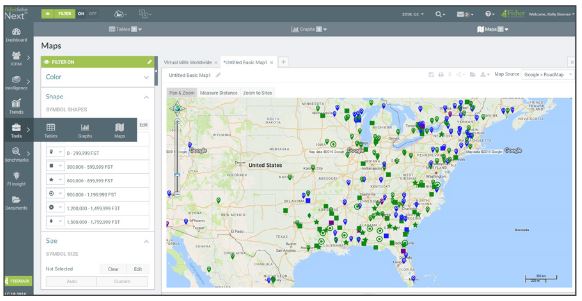The image showcases a webpage dedicated to map visualization and customization. Dominating the interface is a large, detailed map of the United States, peppered with multicolored pinpoints, including green, blue, and purple markers indicating various locations or data points. At the top of the page is a grey navigation bar containing several icons, such as a magnifying glass for search functionality and an envelope indicating mail or messages. Alongside these, there's a set of account settings icons facilitating user customization.

Beneath this bar lies a prominent green button labeled "Filters," which appears to be activated. Adjacent to this is a filter section distinguished by a green background, offering a diverse array of filter categories like color, shape, and size. These filters come with dropdown menus that enable users to fine-tune the map's display according to their preferences. The right side features additional interactive icons and customization options, making the webpage highly interactive and user-friendly. The backdrop of the map highlights prominent geographic features, including the expansive Atlantic Ocean to the east.